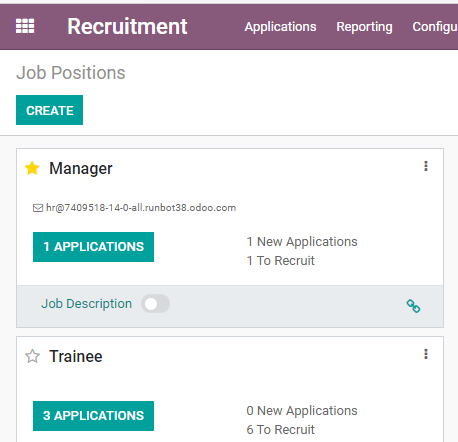Detailed Caption:

This image is a smartphone screenshot of a website named "Recruit." The interface features a light purple border with a grid of nine squares followed by the word "Recruitment." Below the header, there are tabs labeled "Applications," "Reporting," and "Configuration." 

In the main white section of the page, the title "Job Positions" is prominently displayed. Directly beneath this title is a green button with white text that reads "Create." Further down, another white section features a yellow star icon next to the title "Manager." To the right of "Manager," there are three vertical dots indicating a menu.

To the left and below "Manager," there is an envelope icon with text next to it which displays, "Our HR at 740-9518-14-0-all-robot38.odoo.com." Adjacent to this text, a button reads "One Application," next to which there is further text stating "One New Applications." Below this, additional text indicates "One to Recruit" followed by "Job Description." There's also a toggle button for "Job Description," which is currently off, along with a link to the right of it.

Subsequently, the next job position listed is "Trainee," marked by a star icon that is not selected. To the right of "Trainee," there are again three vertical dots for a menu. Directly below the "Trainee" title, a green button with white text indicates "Three Applications." To its right, the text reads "Zero New Applications," and below this, "Six to Recruit" is noted.